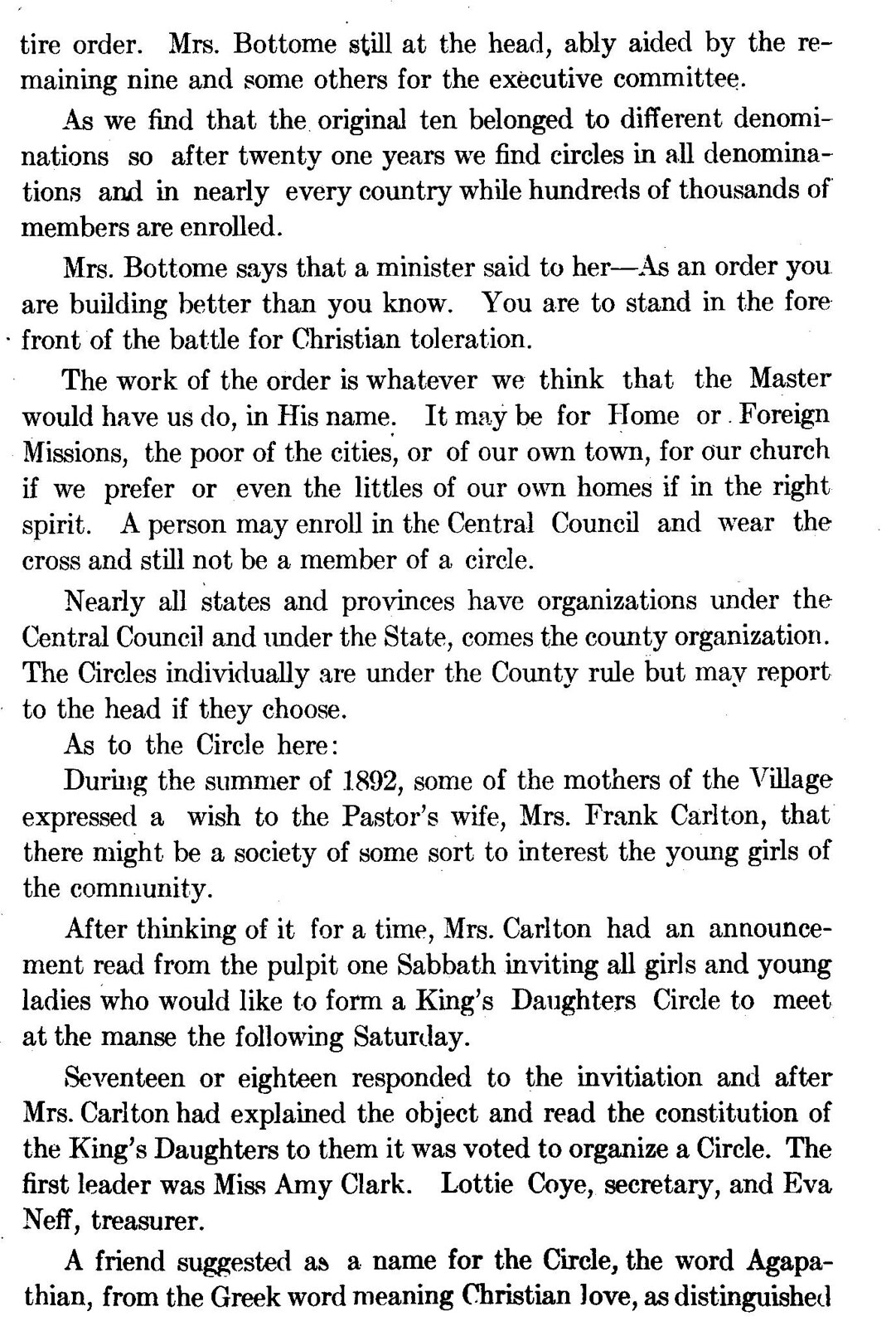This image shows a page from a book with black text on a white background, giving it a transparent appearance. The text begins mid-sentence with "tire order," followed by: "Mrs. Bottom is still at the head, ably aided by the remaining nine and some others for the executive committee. As we find that the original ten belong to different denominations, so after 21 years, we find circles in all denominations and in nearly every country while hundreds of thousands of members are enrolled. A minister said to Mrs. Bottoms, 'You are building better than you know. You are to stand in the forefront of the battle for Christian toleration.' The work of the order includes various activities thought to be aligned with the master's wishes, whether for home or foreign missions, the poor of cities or towns, their church, or even the welfare of their own homes. Nearly all states and provinces have organizations under the central council, and individual circles may choose to report directly to the head. In the summer of 1892, mothers in a village expressed a desire for a society to interest young girls, leading Mrs. Frank Carlton, the pastor's wife, to invite potential members to form a King's Daughters Circle. After receiving 17-18 responses, and following Mrs. Carlton's explanation of the objectives and constitution, the circle was organized with Miss Amy Clark as the first leader, Lottie Coy as secretary, and an individual named Eve as treasurer. A friend suggested naming the circle 'Agapithaeon,' derived from a Greek word meaning 'Christian love as distinguished.'"